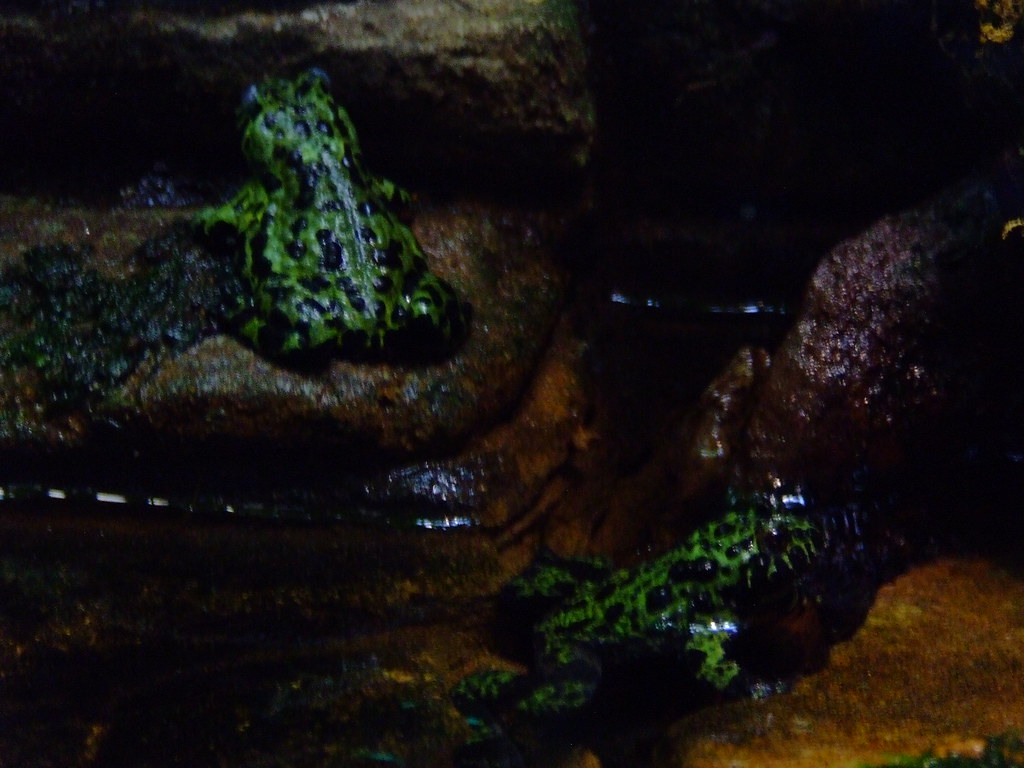The image features two vibrant neon green frogs with dark spots, situated in a wet, rocky area that is dimly lit. The scene includes a small pool of water and multiple rocks, all appearing slick and wet. The frog on the top left sits on a damp rock, with its back facing the camera. The rock on which it rests has patches of green algae. Toward the lower part of the image, the second frog is partially submerged in the pool, extending out toward the rocks. The rocks, predominantly dark brown, show signs of algae or potentially mold, adding texture to the scene. The bright coloration of the frogs suggests an exotic or possibly poisonous nature, enhancing the captivating nature of the photograph likely taken in a controlled environment, such as a tank.